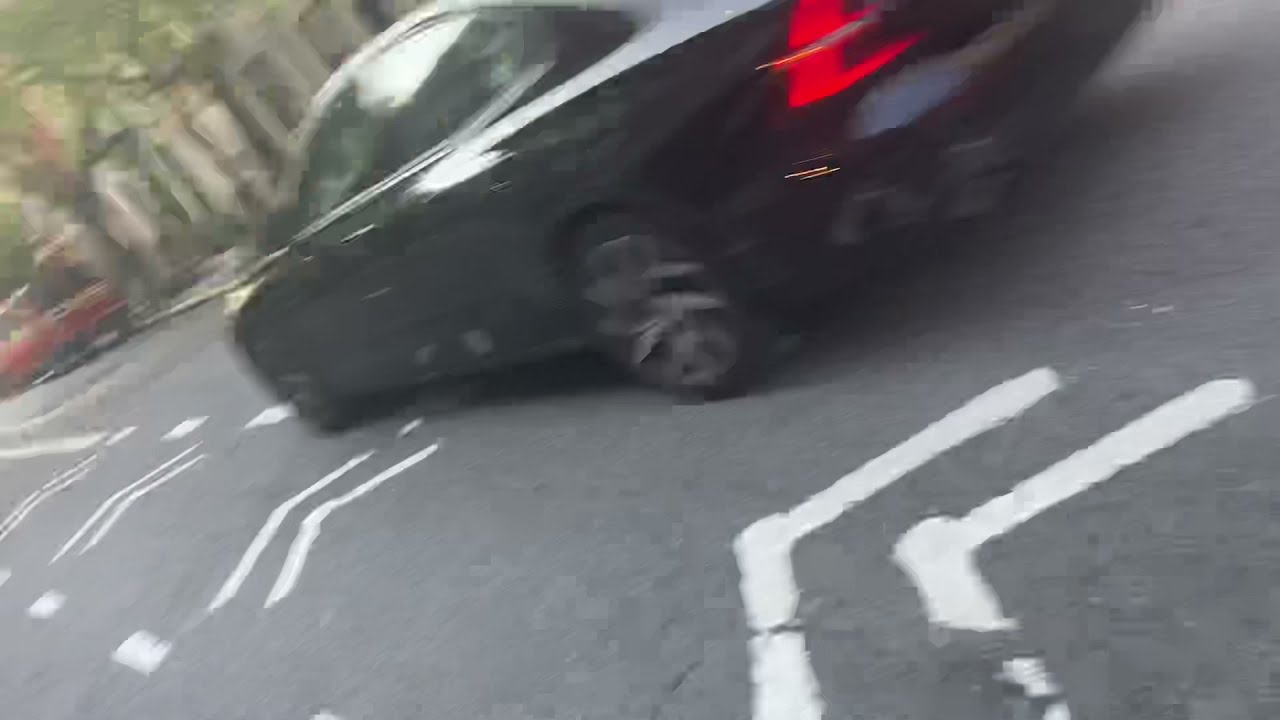The image depicts a slightly blurry scene of a black sedan moving down a residential street in a downtown area during the daytime. The car, captured at an angle from an upper viewpoint, has its red brake lights illuminated, indicating it might be braking. The street is paved with blacktop and adorned with worn white arrows and dotted lines. On the left side of the car, the road markings are visible. In the background, to the right of the sedan, there are houses and a sidewalk where a red vehicle is parked. Further into the distance on this side, a large tree with full green foliage stands next to the red vehicle. Additionally, a person can be faintly seen on the far left side of the image. Light reflections off the black car's body and wheels further emphasize its motion, while the overall blurriness adds a sense of dynamic movement to the scene.